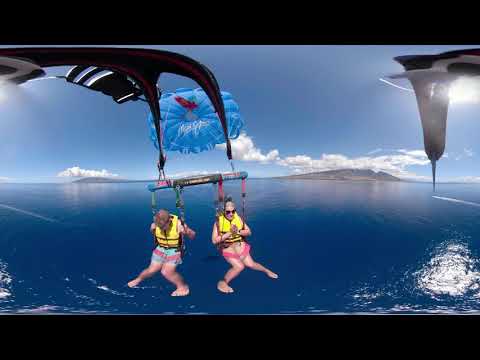The image captures a wide-angle shot of two individuals engaged in a water sport, suspended beneath a hang glider-like apparatus over a vast expanse of serene, dark blue ocean. Both individuals are securely seated in harnesses, behind which a white parachute with a distinctive red streak and indiscernible white lettering is fully deployed. The parachute is connected to a larger black arm extending from the apparatus. 

The individuals, adorned in yellow life vests and colorful swimsuits—one wearing blue and pink striped shorts and the other in pink shorts—each adopt a similar pose with their thighs together and legs extended outward in an 'A' shape. One person, on the left, glances down at the water, while the other, on the right, wearing black sunglasses, looks ahead with arms positioned in front of their chest. 

The background features a clear, bright blue sky with minimal cloud coverage, while the calm water below is a striking blue without any visible waves. In the far distance, small and large islands dot the horizon. The top right corner of the image is slightly obstructed yet illuminated by the sun.